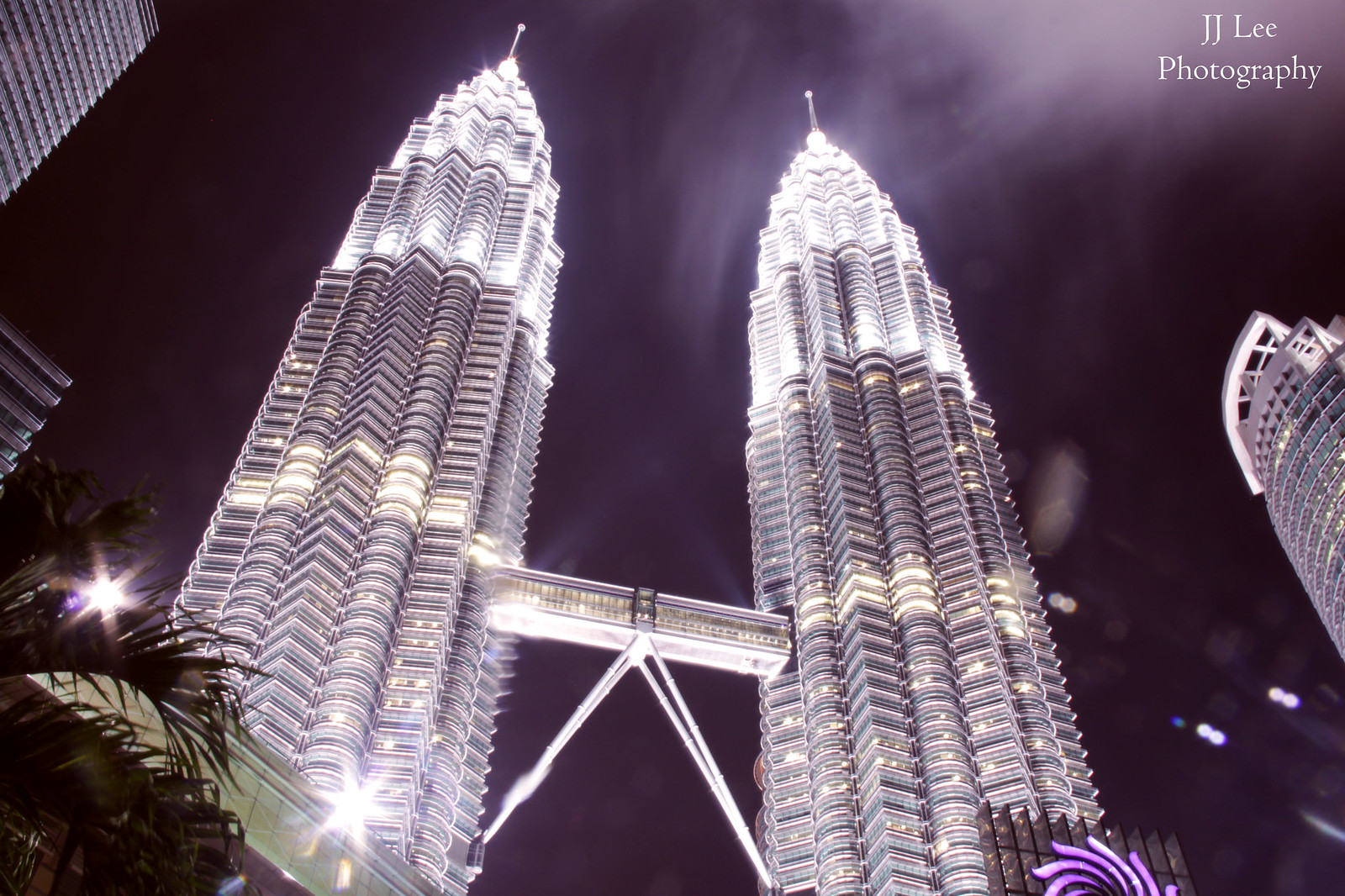This nighttime photograph, taken from the ground looking up, showcases the iconic Petronas Twin Towers with their stunning architectural design resembling crinkled cupcake papers or missiles due to the progressive narrowing and textured detailing of their multiple stories. Each tower is brightly illuminated, with the lights creating a sparkling effect against the dark, slightly cloudy night sky. Midway up, a connecting walkway, also brightly lit, bridges the two towers. In the lower left, palm fronds are visible, while the edges of other buildings appear on the left and bottom right of the frame. Additionally, a cylindrical building with many stories is partially seen on the middle right. The top right corner of the image bears the text "JJ Lee Photography."